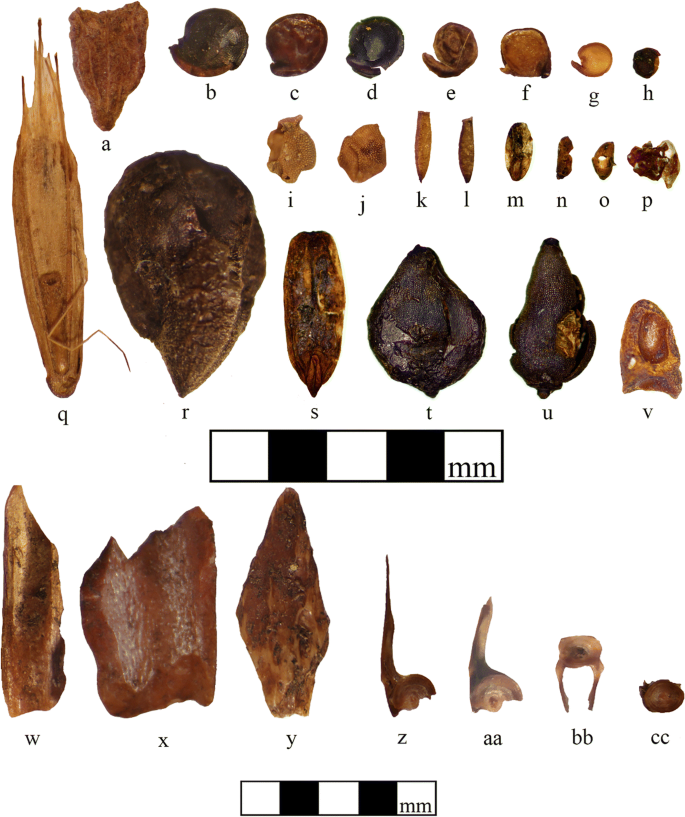This detailed image against a plain white background without visible borders showcases a carefully arranged collection of 29 archaeological artifacts, likely originating from the American West or Southwest. The artifacts, possibly ancient tools or arrowheads, are arranged in a grid format with labels ranging from lowercase letters A to Z and continuing with double letters A, A, B, B, and C, C. They vary significantly in shape and size, with some being very tiny and others relatively large. The items appear predominantly in dark brown to black hues, with some lighter gray ones among them.

The artifacts' arrangement starts from the top left corner and proceeds to the right in rows, spanning four rows in total. The items labeled A to P seem to be decreasing in size, resembling pebble-like forms. The artifacts labeled Q to R are among the largest, whereas S through V progressively reduce in size. W, X, and Y are again relatively large, invoking the impression of arrowheads. The last set, labeled Z, A, A, B, B, and C, C, includes objects of indeterminate shapes that could be small bones or other miscellaneous items.

A checkered black and white scale, marking millimeters, is centrally placed for size reference, with no explicit labels indicating their exact measurements. This image, lacking detailed captions and specific origins, remains an ambiguous yet intriguing visual catalog of these ancient artifacts.